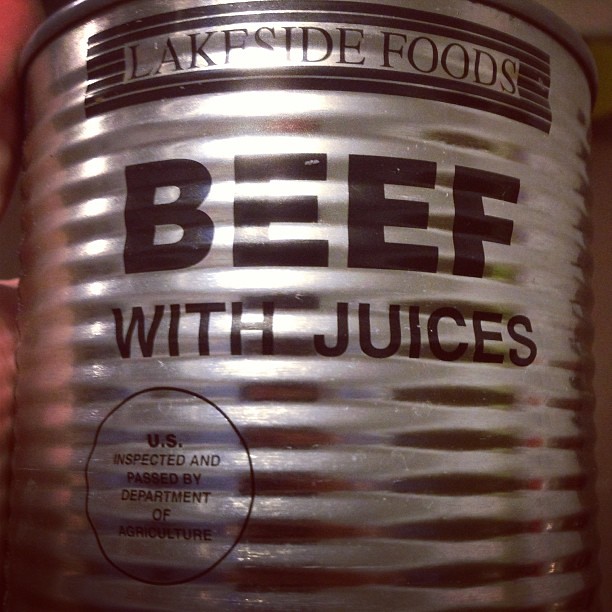This image is a close-up, slightly blurry, color photograph of a ribbed silver metal can, possibly aluminum, with distinctive highlights and shading across its horizontal grooves. Prominently displayed at the center of the cylindrical can are the bold, black letters spelling "Beef," followed immediately below by smaller black text reading "with juices." At the very top of the can, there's a horizontal label wrapped around it within a dashed black box, stating "Lakeside Foods." On the lower left corner, a black circle contains the words "U.S. inspected and passed by Department of Agriculture." There is a subtle pinkish hue reflecting off the left side of the can, with a slight greenish tinge towards the right. Additionally, the background features what appears to be a red section, possibly a wall or cabinet. The can’s textured surface and the interplay of light make the image particularly striking.